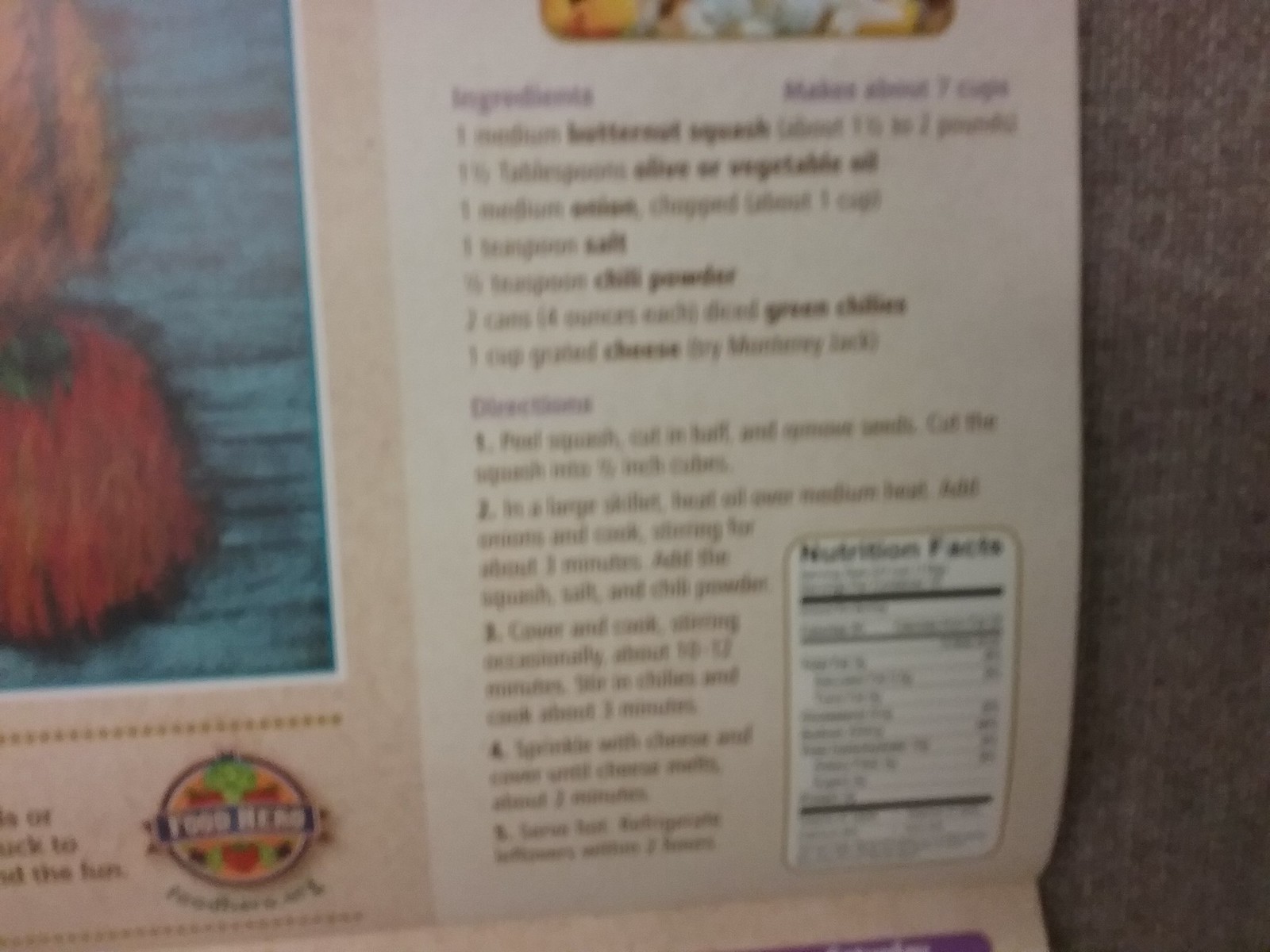This very blurry photograph appears to be the back of a food packaging, featuring a recipe along with nutritional facts located in the bottom right corner. At the top left, there is an illustration of the prepared dish. The recipe, positioned in the middle of the image, provides a list of ingredients for a soup that yields approximately 7 cups. Although some text is unclear, the visible portions mention adding one medium butternut squash and one and a half teaspoons of olive or vegetable oil.